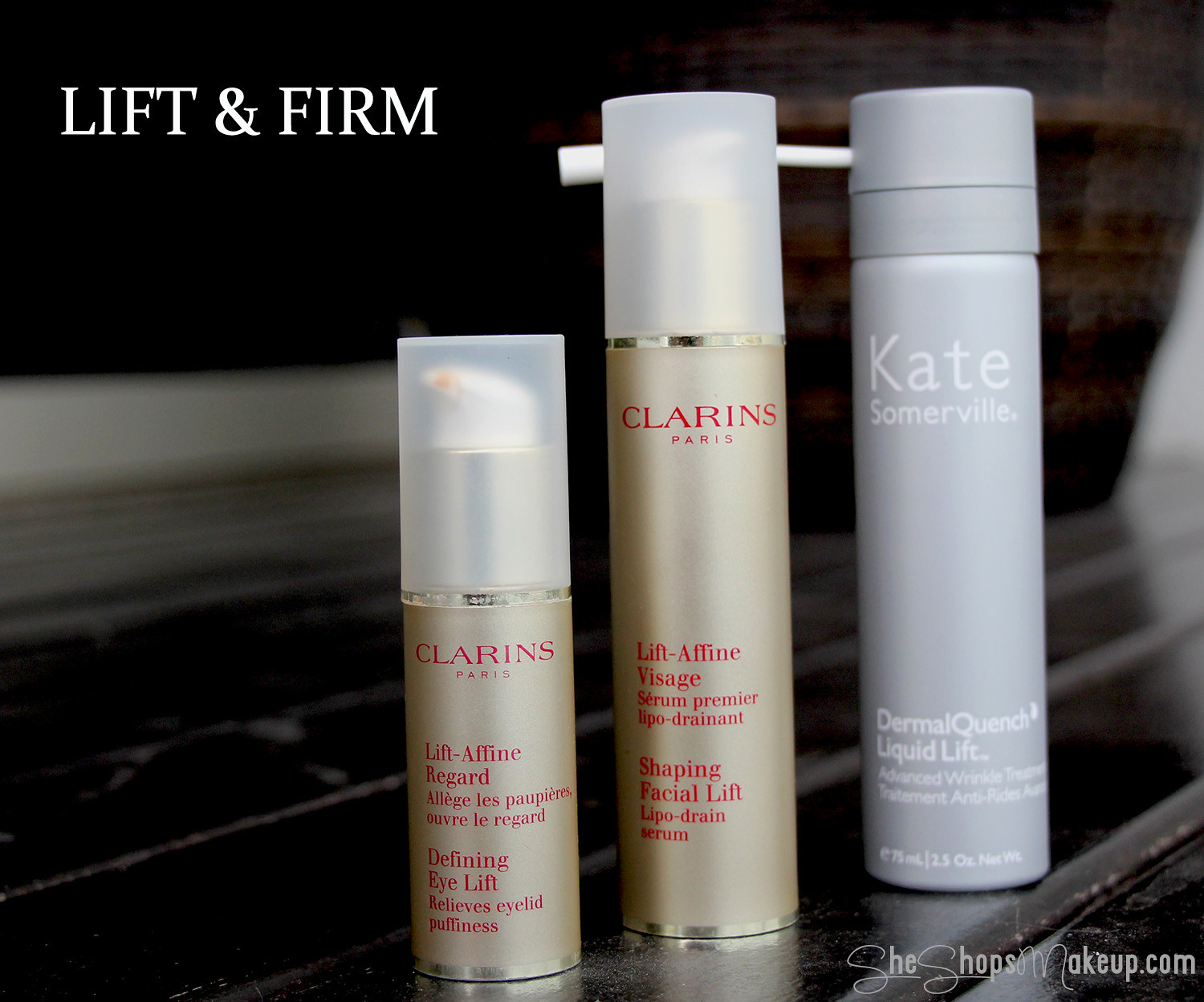This advertisement showcases three premium skincare products against a predominantly dark background, which features a blend of black, gray, and white hues. In the top left corner, bold white capital letters spell out "LIFT & FIRM." The products are meticulously arranged on what appears to be a shiny gray or black surface. 

From left to right, the first product is the smallest in height. It's a light beige metallic tube labeled "Clarins Paris." The product name, "Lift Affine Regard," followed by French text, and the description "Defining Eyelift" below, indicates it relieves eyelid puffiness. Next, the middle product is another tan-colored tube from "Clarins Paris," taller than the first. It bears the name "Lift Affine Visage," again followed by French text, and the translated description "Shaping Facial Lift Lipo-Drain Serum" at the bottom. Both Clarins products feature red lettering and clear lids, revealing white pumps underneath.

The third product is distinctively different in color and brand. It’s a grey cylindrical bottle with a white pump, marked with "Kate Somerville" in large white print. Below this, it states "DermaQuench Liquid Lift," followed by additional but unreadable text.

In the bottom right corner of the image, the text "SheShopsMakeup.com" is subtly inscribed, adding a final touch of detail to this elegant cosmetic display.